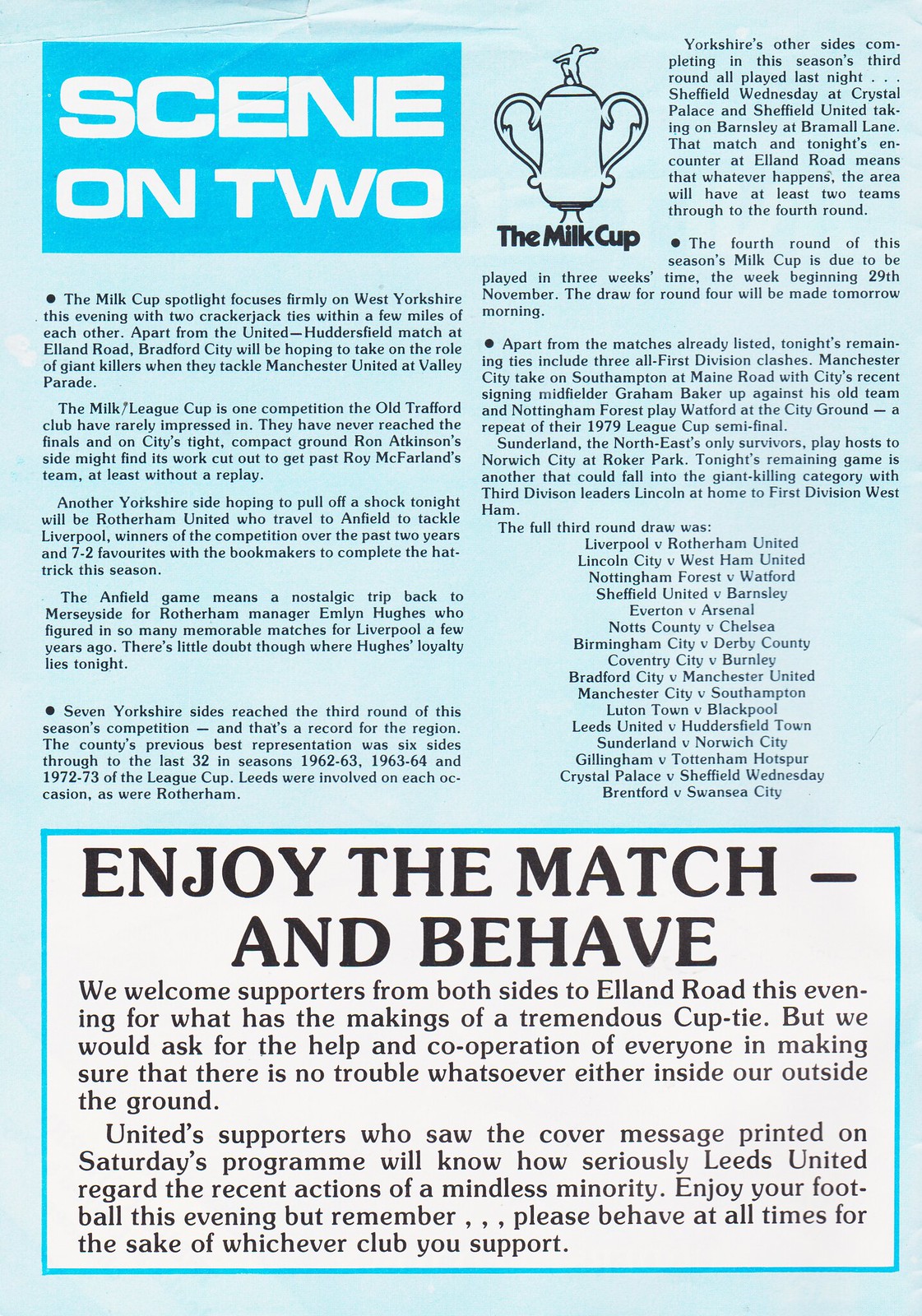The image is a page from a program about the English football event, specifically the Milk Cup. The page features a turquoise background and is formatted with two columns of text. In the upper left corner, there's a blue box with white text that reads "Seen on 2". The main content discusses highlights of upcoming Milk Cup matches, focusing on teams from West Yorkshire, including detailed descriptions of significant fixtures such as Bradford City vs. Manchester United at Valley Parade, and Rotherham United vs. Liverpool. These descriptions highlight the competitive nature of the games and historical contexts. Towards the bottom of the page, there is a white box with a blue border titled "Enjoy the Match and Behave", which contains instructions for the audience and sportsmanship guidelines. This section also features a line drawing of the Milk Cup trophy, emphasizing the significance of the competition.